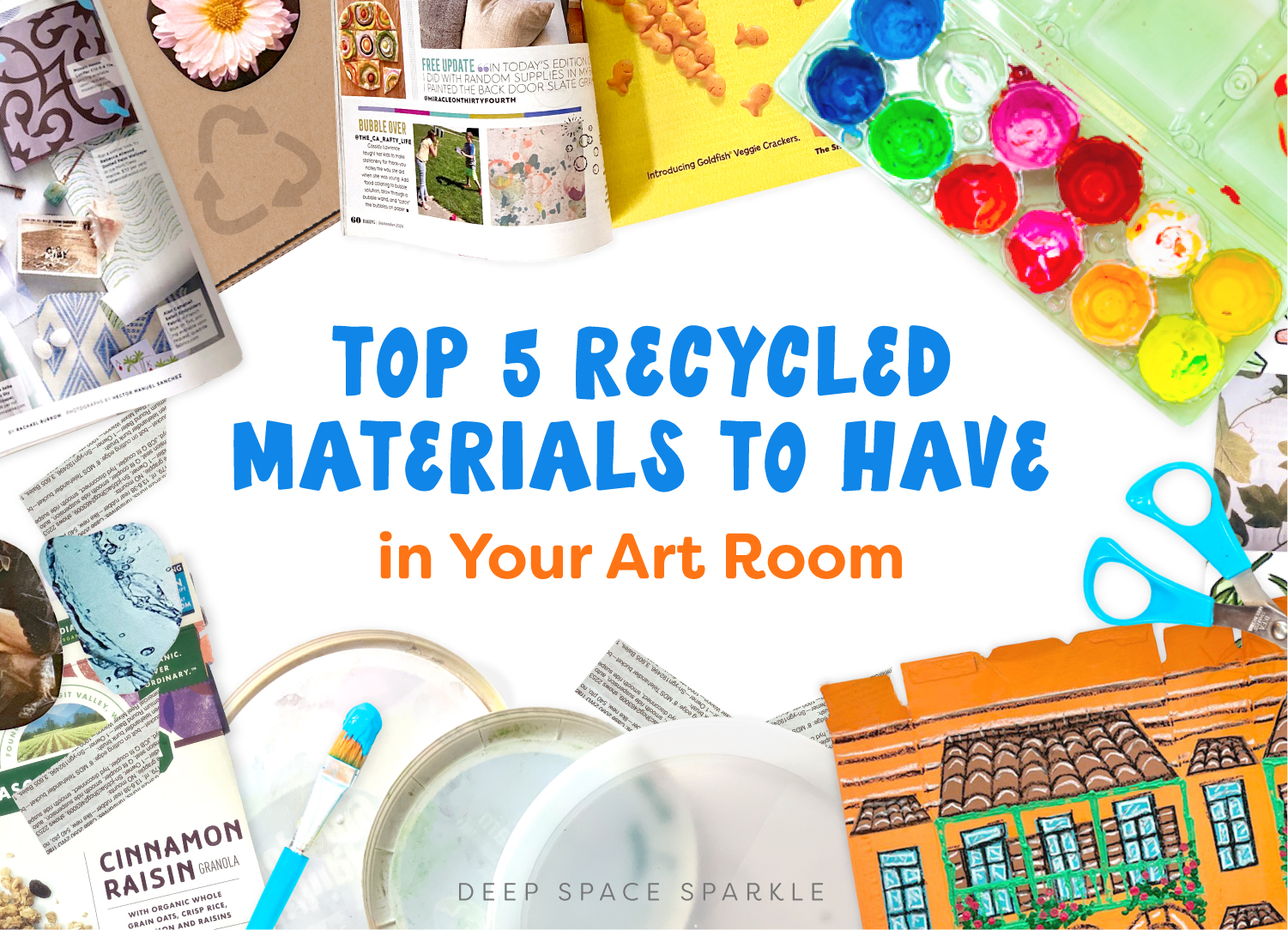Centered on a crisp white background, this promotional material prominently features vibrant blue text reading "Top 5 Recycled Materials to Have." Just below, bold orange letters declare "In Your Art Room," making the theme clear. The design is intricately bordered with an array of eclectic, detailed graphics, beginning with the bottom left corner.

In this section, a magazine page fragment showcases the phrase "Cinnamon Raisin" alongside an organic whole grain oats description in black ink, partially obscured with white space and further adorned with torn magazine images. Ascending upward, a torn paper strip, possibly from a publication, intersperses with more magazine snippets.

To the right of this collage-like composition, a prominent brown piece of paper features a recycling symbol in a darker shade, crowned by an illustrated flower. Nearby, an open magazine displays on its left page a detailed article, while the right page bursts with yellow hues, introducing "Golden Veggie Crackers" in challenging-to-read text.

Further right, an assortment of colorful paints — blue, green, red, pink, yellow, and differing yellows — are featured, topped with shades of white, red, pink, aquamarine, and teal, set against a striking backdrop. Adjacent to this palette, a pair of scissors with a light blue handle is neatly positioned.

Beneath the scissors, a charming crayon drawing depicts a terracotta home with a tiled roof, verdant plants adorning the windows, and five visible windows, adding a whimsical touch. To the left, paper plates and more torn text complete this creatively cluttered and vibrant border, encapsulating the spirit of recycling and artistic inspiration.